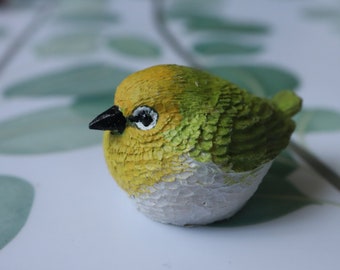The photograph showcases a detailed, miniature sculpture of a plump, ceramic bird with a golf-ball-like round shape. The bird's head is an orange-ish yellow with a mustard tinge, its beak is black, and its eyes are black encircled by white and black rings. The bird's chest transitions to a vibrant yellow, while its back, wings, and tail display varying shades of green, from lime to dark olive. The belly of the bird is white. Notably, the texture of the wings is meticulously crafted, revealing individual feathers. The bird sits atop a white surface, possibly a tablecloth, adorned with a green leaf and brown branch pattern. This vividly covered background is slightly blurred, ensuring the colorful and intricately designed bird remains the focal point of the image, positioned slightly to the right of center.